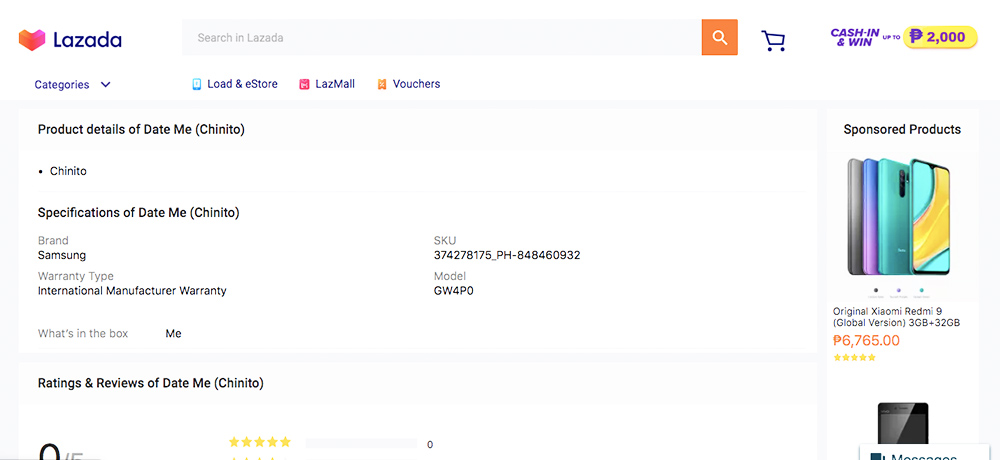The screenshot captures the interface of the Lazada app. In the upper left corner, a 3D hat icon in pink is visible, symbolizing a special feature or category. Positioned to the immediate right of the hat icon is the brand name "Lazada." Following the branding, there's a search bar with a distinct orange search icon beside it. Further along the top right, there's a shopping cart icon.

Below the word "Lazada," on the left side of the screen, there is a dropdown menu for categories. Underneath the categories dropdown, in black text, it states "Product details of date May. Chinito."

On the right side of the image, four colorful smartphones are arranged side by side. Below these smartphones, also in black text, is the label "Original Xiaomi Redmi 9." Additionally, a promotional banner written in purple offers a chance to "cash in and win up to $2,000."